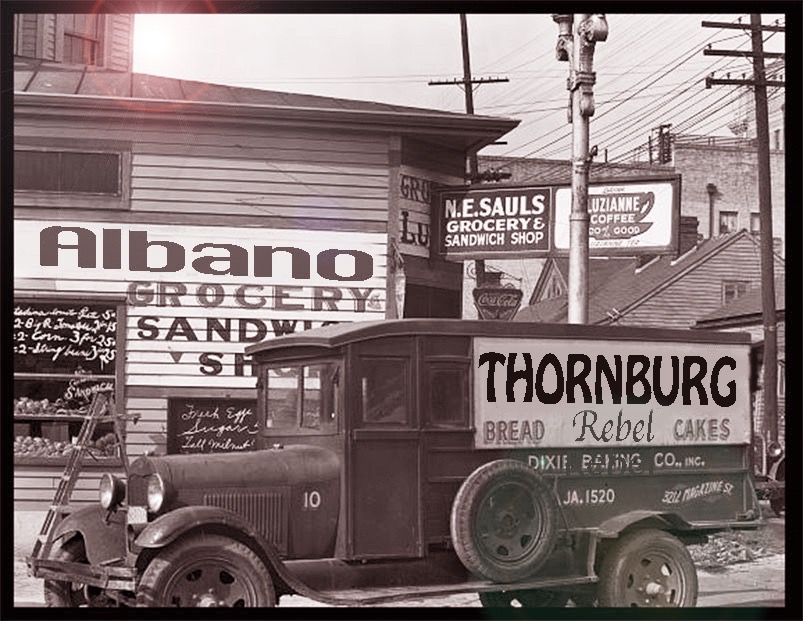This is a detailed horizontal rectangular black-and-white photograph with numerous shades of brown, capturing a scene from the early 1900s to the late 1930s or early 1940s. In the foreground, an old delivery truck prominently features signage that reads "Thornburg Bread Rebel Cakes." The truck, marked with a triangular device on the front grill and a spare tire behind the front door, has additional text on the side mentioning "Dixie Parking Company Incorporated."

The truck is parked before a series of shops. To the immediate right, a wooden clapboard building with a roof and windows is labeled "Albano Grocery Sandwich Shop" on a white sign with black letters. Adjacent to this store, another establishment displays "N.E. Saul's Grocery and Sandwich Shop." The shop windows bear handwritten notes in white, detailing items for sale.

In the upper left of the background, telephone poles with wires running in multiple directions add a historical ambiance. The upper right features more signage, including one for "Louisiana Coffee," along with visible rooftops and the upper parts of additional buildings. The meticulous arrangement of elements enhances the vintage charm and storytelling of the image, inviting viewers to glimpse life from a bygone era.